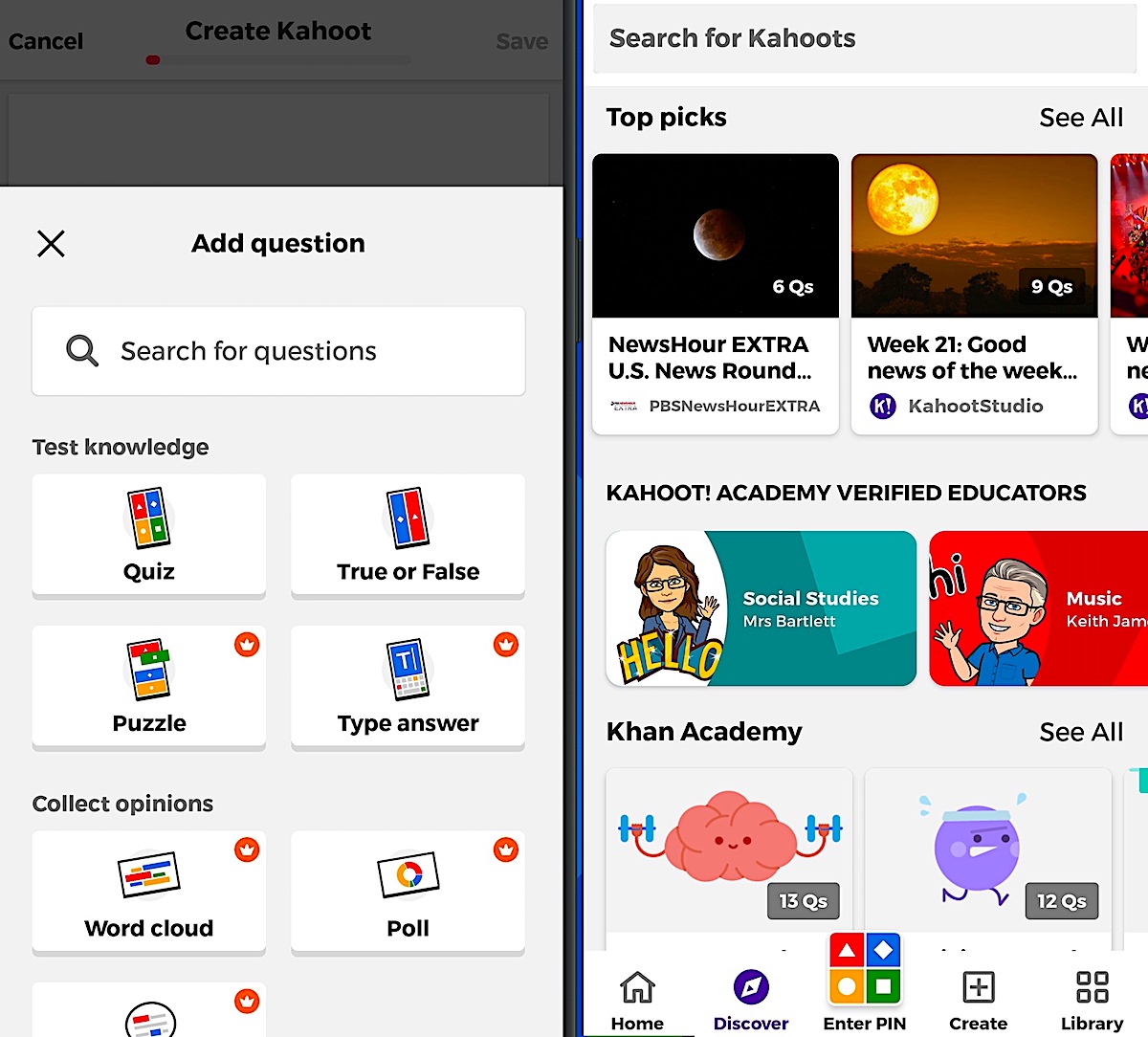The image shows two adjacent screens. The left screen displays an interface with a grayed-out film strip along the top. Below this strip is a button labeled "Cancel" and another labeled "Create Kahoot" (spelled K-A-H-O-O-T). Below these buttons, there is a status bar with a small section of the bar filled with red on the left, while the rest is gray. Towards the lower portion of the screen, there's a pop-up box displaying an 'X' in the top-left corner, with the text "Add Question" prominently underneath.

Further down, there's a search bar labeled "Search for Questions." Beneath this, the screen lists several options including "Test Knowledge" with corresponding buttons for different types of questions: Quiz, True or False, Puzzle, Type of Answer, Collect Opinions, Word Cloud, and Poll. The last option is partially cut off.

The right screen features a search bar titled "Search for Kahoots." Below this, there's a section labeled "Top Picks" with an option to "See All." This section highlights various educational themes such as "News Hour Extra," "U.S. News Round," "News Week 21," and "Good News of the Week." Further down, there's a section titled "Kahoot Academy" featuring categories like "Verified Educators," "Social Studies" by Ms. Bartlett, "Music" by Keith James, and "Khan Academy." 

The screen also contains visual elements like an image of a brain lifting weights, representing 13 questions, and a purple circle depicting someone running, indicating 12 questions.